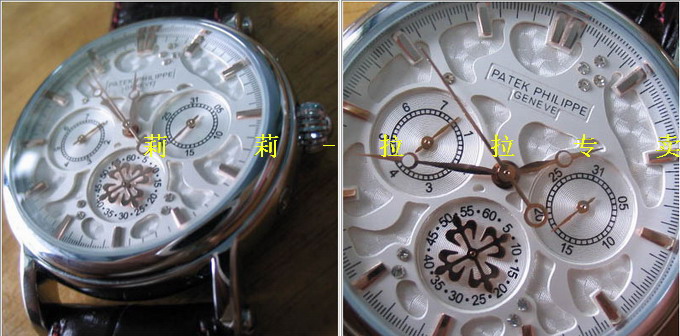Side-by-side images showcase an elegant yet possibly counterfeit Patek Philippe watch, drawing attention with its rose gold detailing on the watch face. The prominent Patek Philippe Genève branding is visible, a name synonymous with luxury and favored by celebrities. The watch face, predominantly white, is adorned with diamond-like gemstones, adding a touch of opulence. Yellow Chinese characters overlay the top of both images, hinting at an Asian market or seller, possibly casting doubt on the watch's authenticity due to its otherwise cheap appearance.